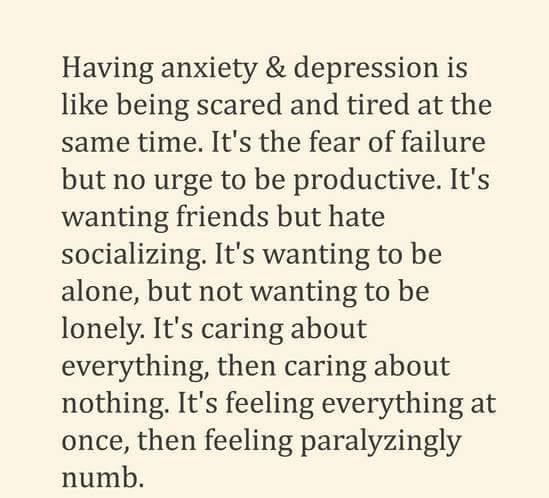The image features a column of black text on a tan background. The text, presented in a standard font, reads: "Having anxiety and depression is like being scared and tired at the same time. It's the fear of failure, but no urge to be productive. It's wanting friends, but hate socializing. It's wanting to be alone, but not wanting to be lonely. It's caring about everything, then caring about nothing. It's feeling everything at once, then feeling paralyzingly numb." The text is centered and takes up most of the image, which has a simple design with no other significant elements. The first letter of each sentence is capitalized, and there is a white border framing the text, giving it a structured appearance.